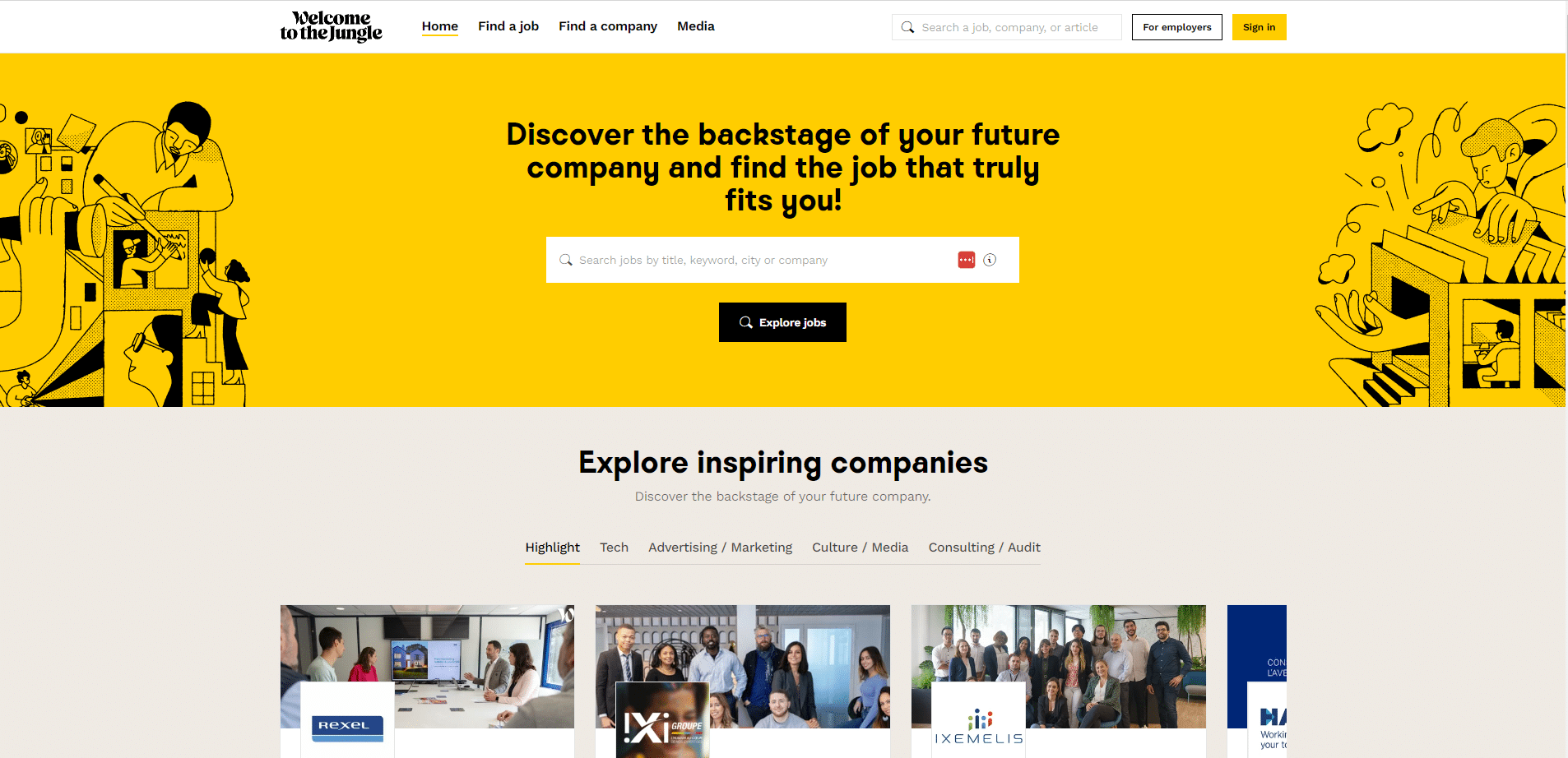The screenshot features a well-organized website interface with a predominant white background. At the top left, in bold black text, are the words "Welcome to the Jungle". To the right of this welcome message, there are navigation options labeled "Home", "Find a Job", "Find a Company", and "Media", with "Home" underlined in yellow indicating it is the currently selected page. 

On the far right side of the header, a white search bar with faint gray placeholder text (though its content is indiscernible) is positioned. Adjacent to the search bar, there is a black square containing the text "For Employees" in black. Next to it, a yellow button with black text reads "Sign In".

Below the header, a prominent yellow banner sprawls across the page. To the left of this banner, a collection of stylized illustrations can be seen. On the right side of the banner, a sketch shows a character navigating through a machine in a crudely drawn yet appealing artistic style.

At the center of the page, in large black text, the heading declares, "Discover the backstage of your future company, and find a job that truly fits you." Beneath this heading sits a white search box with a magnifying glass icon next to it. A smaller black rectangle just below the search box contains white text that reads "Explore Jobs".

Further down, a section with a gray background and black text invites users to "Explore Inspiring Companies". Additional gray text is present in this area, though the specifics are unclear. Three simplistic logos depicting business-themed illustrations complete the visual elements, emphasizing networking and professionalism.